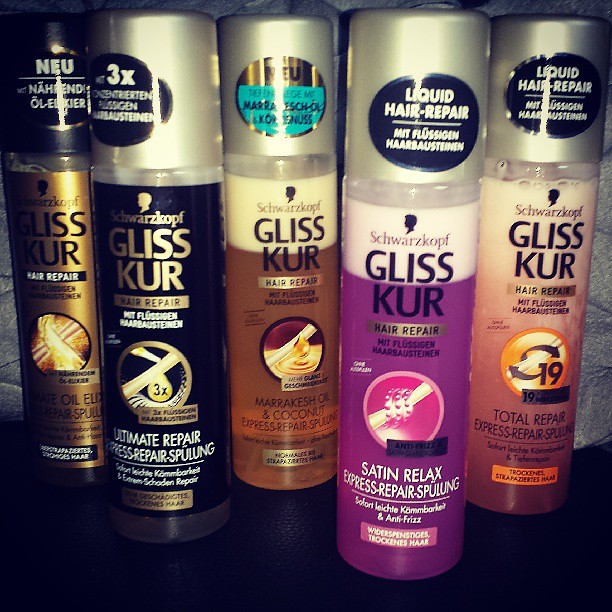This color photograph displays a lineup of five cylindrical bottles of Schwarzkopf's GLISSKUR hair repair products. Each bottle is uniquely colored and labeled. From left to right:

1. The first bottle features a gold banner reading "Hussur Hair Repair," with a partial view of the word "Neuhand Ole Kier." There's an illustration of a close-up hair root below.
2. The second bottle is black and labeled "Ultimate Repair." It emphasizes "3x Repair Power" with a graphic depicting triple-action repair.
3. The third bottle, containing amber-colored liquid with a white top, is labeled "Marrakech Oil and Coconut Express Repair Serum" and showcases a cream image.
4. The fourth bottle has a purple bottom transitioning to white at the top and reads "Satin Relax."
5. The final bottle has a peach-colored bottom and a white top with the label "Total Repair."

All bottles are lined up in a single file, representing variations of the GLISSKUR hair repair range, denoted by their distinct colors and specific repair formulas.